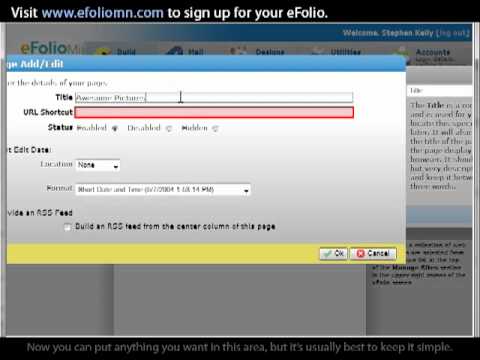A screen capture from a computer monitor featuring the website efoliomn.com with a banner across the top that reads "Visit efoliomn.com to sign up for your eFolio." The main content of the webpage is obscured by a pop-up window, making the underlying site barely visible. In the upper left corner of the pop-up window, a blue bar displays the text "Add" followed by an indistinct blur, possibly "slash" and "DIT." 

The pop-up window appears to be a form titled “Details of your page.” Directly below, there is a text box labeled "Title," with someone actively typing into it, though the text entered is unreadable due to blurriness. Next, there is a label "URL Shortcut" with an empty text box highlighted in red. Further down, the label "Status" is visible but too blurry to discern the available options. 

A subsequent label, "Date," is partially legible, accompanied by a dropdown menu showing "None." Underneath this dropdown, there is a longer, blurred text box that likely contains date and time information. The next section appears to instruct the user to "Provide an RSS feed," with a checkbox and the option "Build an RSS feed from the center column of this page."

At the bottom of the pop-up window, there is a yellow banner with two buttons: "OK" on the left and "Cancel" on the right. The content behind the pop-up window remains indistinct and unreadable, contributing to the overall obscurity of the scene.